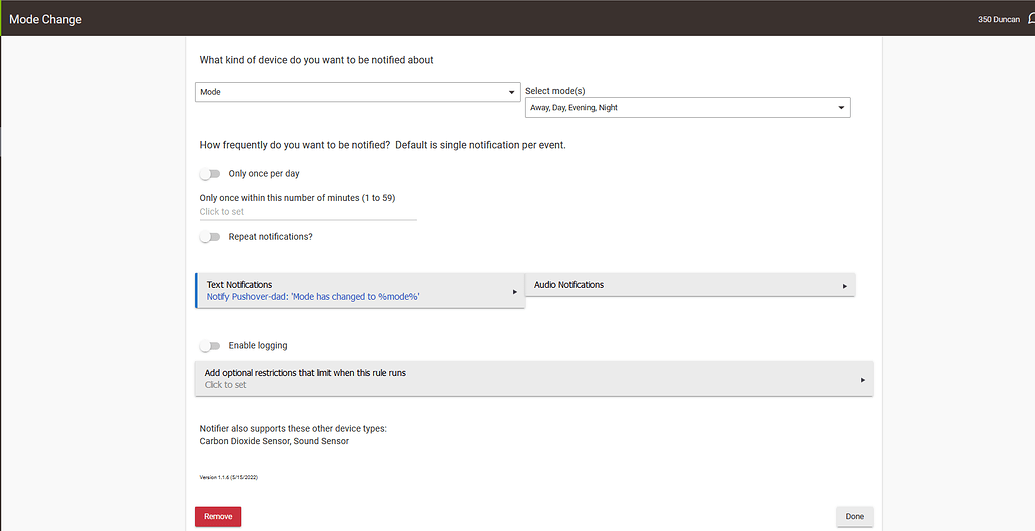The image features a webpage with a black box titled "Mode Change" prominently displayed across it. In the center of the website, there's a section asking, "What kind of device do you want to be notified about?" Below that, a dropdown menu labeled "Select Mode" offers options such as Away, Day, Evening, and Night for users to choose from.

Further down, the page prompts, "How frequently do you want to be notified?" The default setting is a single notification per event, with additional options to select frequencies ranging from once within a specified number of minutes (1 to 99). Users are instructed to "Click to set."

The page continues with a query, "Repeat notifications?" and includes gray text that reads, "Notifications, modify pushover." Additionally, there's a note in blue text indicating that a mode has changed, though the exact details are unclear.

An "Auto Notifications" section appears next, followed by an "Enable Logging" option. Gray text here suggests adding optional restrictions to limit when the rule runs, and users are again prompted to "Click to set."

Lastly, the notification settings page mentions that it supports other device types such as carbon dioxide sensors and sound sensors. At the bottom of the page, there's a red box with indistinct white text, making it difficult to discern its contents.